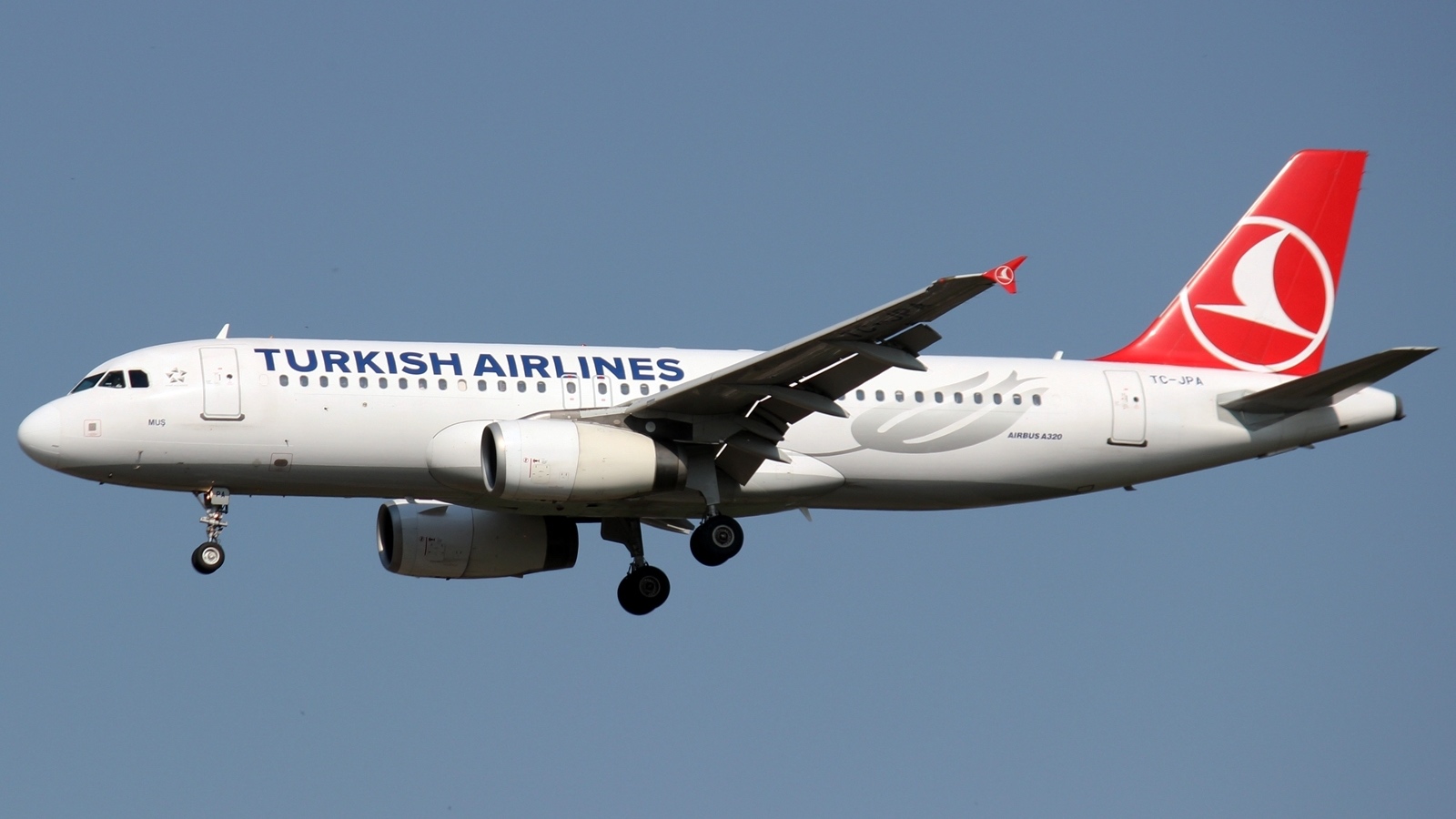This image captures a Turkish Airlines Airbus A320 in mid-flight against a backdrop of clear blue sky, giving an impression that it might have been digitally enhanced. The airplane, prominently centered in the photo, is a sleek, brand-new commercial passenger jet. The aircraft's body is primarily white with a distinct red tail, featuring a white bird logo encased in a circular border. Additionally, the same red and white logo is present on the tips of the wings. Turkish Airlines is inscribed in blue text along the fuselage, and the aircraft’s registration code, TC-JPA, is visible on the tail. The plane’s design includes a series of windows along its side and a stylized gray-silver flower motif towards the rear, further accentuating its modern appearance. The overall clarity of the sky with its uniform blue color and absence of clouds enhances the serene yet majestic portrayal of the aircraft in flight.